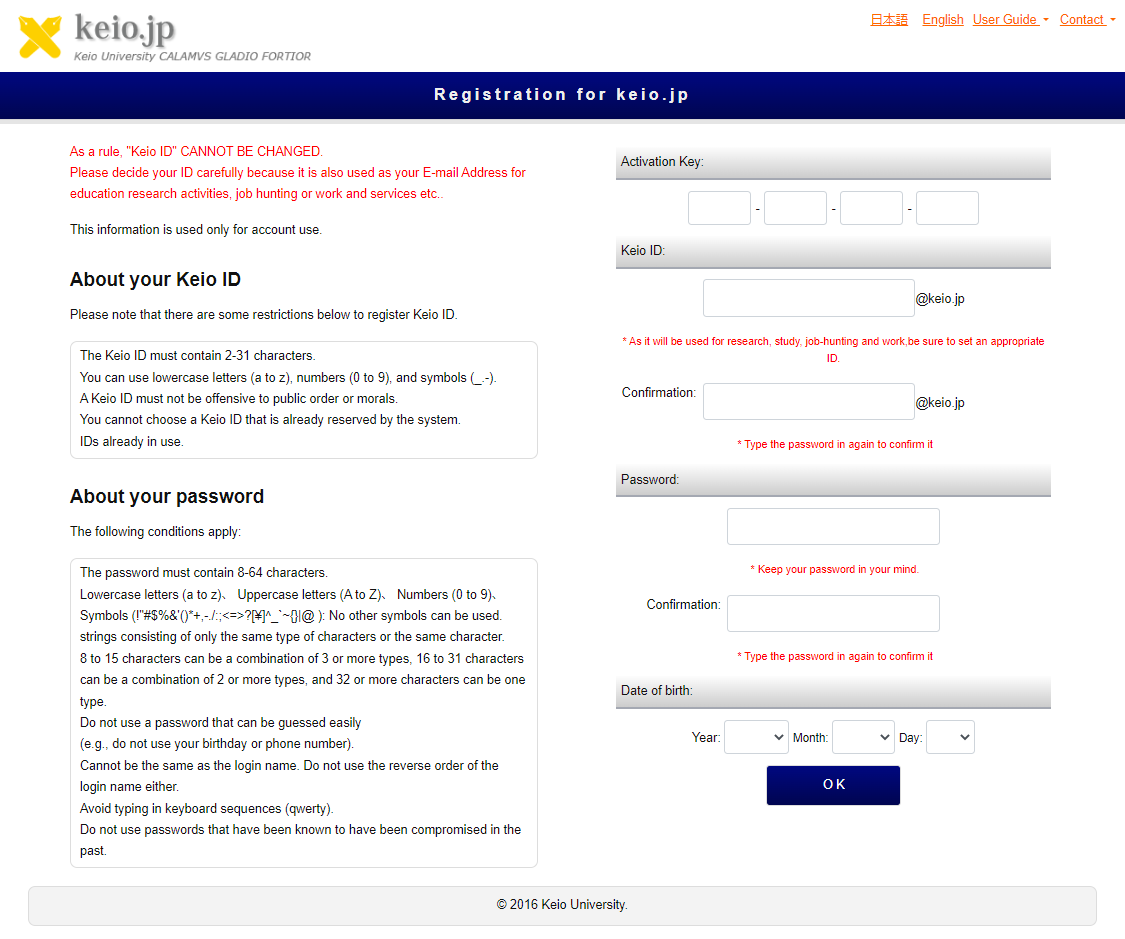The image prominently features detailed instructions for creating and managing a Keio University ID, essential for accessing various educational and research services. At the top, the header reads "keio.jp, Keio University," followed by the Latin phrase "C-A-L-A-M-V-S, G-L-A-D-I-O-F-O-R-T-I-O-R." On the top right, there is some Japanese text, along with links for "English User Guide, Contact, Registration for Keio.jp." 

The main text emphasizes the importance of selecting a Keio ID carefully, as it will be used for email and various academic and professional activities. The Keio ID must be between 2 to 31 characters long, comprising lowercase letters (A-Z), numbers (0-9), and permissible symbols (underscore, hyphen). The ID must respect public order and morals and cannot be already reserved or in use.

For passwords, the requirements are stringent: they must be between 8 and 64 characters and include lowercase and uppercase letters, numbers, and symbols. Passwords should not use easily guessable information like birthdays or phone numbers, nor should they replicate or reverse the login name. Specific combinations and lengths of characters are required, emphasizing strong security practices.

The instructions stress the necessity of setting an appropriate and secure ID and password, with repeated confirmations for accuracy. Supplementary fields include the date of birth (year, month, day), and the image notes that this information is protected under a copyright notice from 2016 by Keio University.